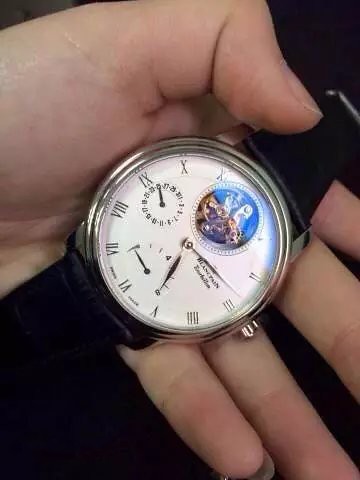The image is a close-up photograph featuring a left hand, likely a lady's given the shape, holding an old-fashioned wristwatch with a black leather strap against a black background. The watch has a silver, circular frame with a white face adorned with Roman numerals. At the top of the face where the 12 would typically be, there's an elaborate cutout revealing the intricate inner mechanics, gears, and small screws of the watch. Thin, gray hour and minute hands indicate a time of approximately 5:13 or 5:14. The watch also includes additional features such as a small inner subdial, possibly indicating the date, and a segment at the bottom with the appearance of an odometer, suggesting it could function as a stopwatch. The name on the watch appears in black writing, likely something Blanc.